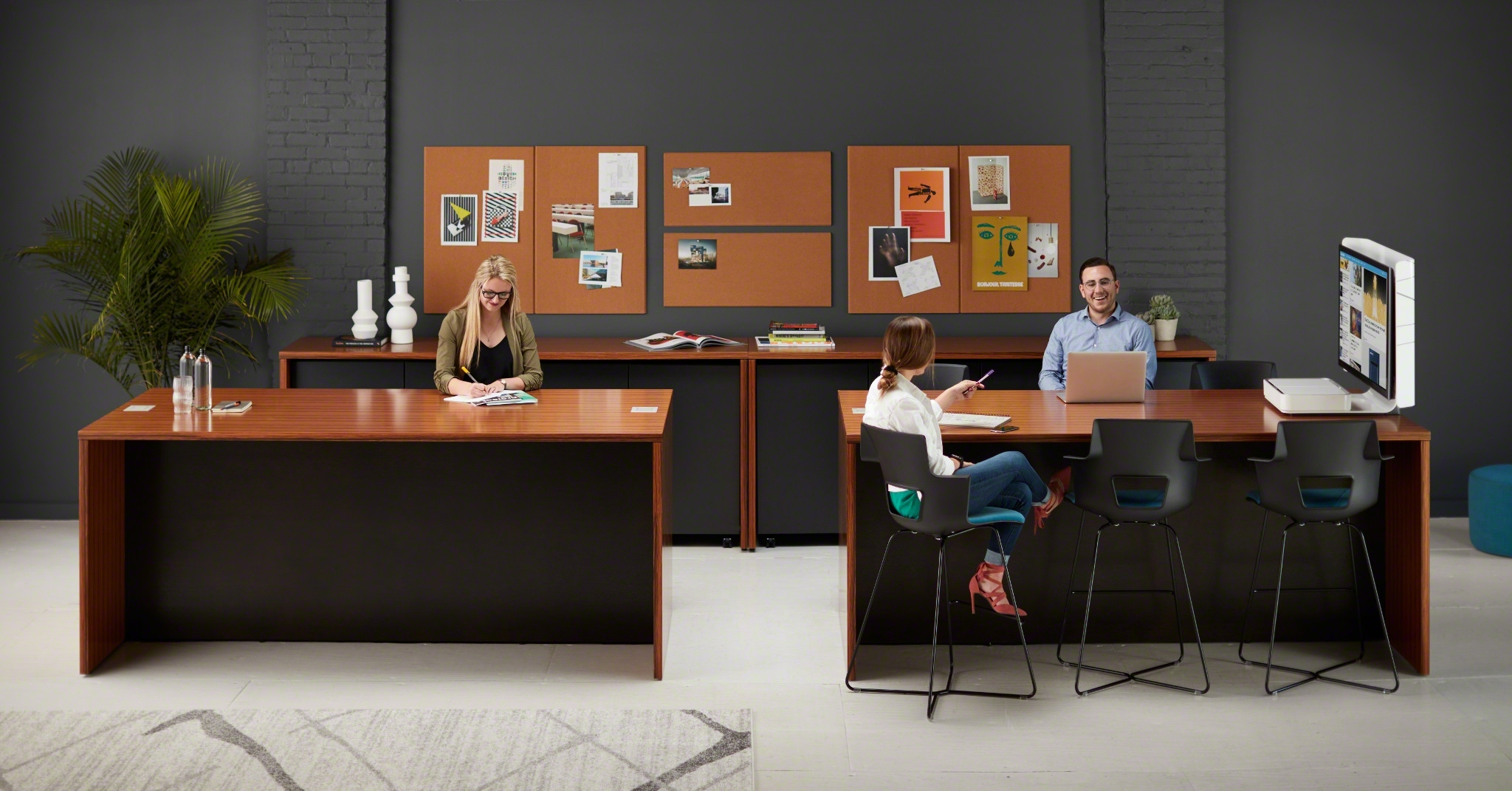In this detailed office scene, the setting features two sleek, medium-shiny wooden desks configured side by side with a small gap between them. The desks sit against dark gray walls with a cream-colored floor. Behind the desks are six pinboards adorned with numerous papers. To the far left, a plant adds a touch of greenery to the space.

On the left desk, a woman with blonde hair is seated facing the camera. She is wearing a green sweater over a black shirt and appears to be writing or drawing, deeply focused on her task. On the desk to the right, a man dressed in a blue work shirt is seated with an open laptop. He is engaged in conversation, smiling towards a woman who is seated on the leftmost of the three black stools in front of his desk. This woman, with brown hair and wearing jeans and a white long-sleeve shirt, has her back to us.

Additionally, the right desk features a monitor positioned next to the man's laptop, adding to the tech-savvy ambiance of the office. The scene exudes a collaborative and interactive environment, characterized by the engaged conversation between the man and the stool-seated woman, contrasting with the focused solitude of the woman at the left desk.